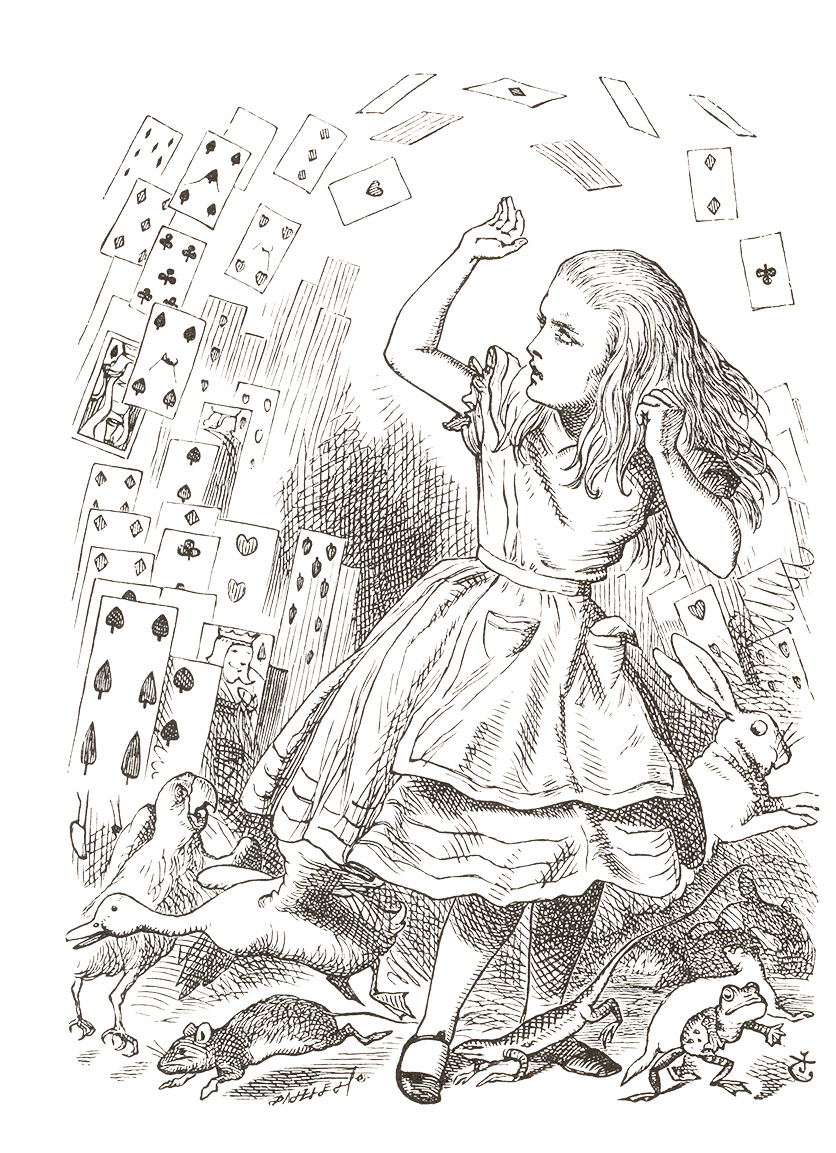This is a detailed black, white, and gray ink drawing depicting a scene from Alice in Wonderland. In the center, a girl with long hair flowing past her shoulders stands dressed in a traditional Alice-style dress with an apron and pockets, complemented by dark ballet slippers. She is positioned in a defensive stance with her hands raised. Surrounding Alice are a variety of animals scurrying around her feet, including a goose, a parrot, a frog, a rat, a reptile, a ferret, a bunny rabbit, and a duck, all appearing frightened and attempting to escape. Above her, playing cards of all suits—hearts, diamonds, clubs, and spades—fly through the air, forming an archway reminiscent of a chaotic rainbow. The detailed cards include the Two of Spades, Two of Hearts, Six of Spades, Queen of Diamonds, Ace of Spades, and Ace of Hearts. Rendered with skill and precision, this monochromatic artwork does not contain any text and is noted for its dynamic composition and intricate shading.